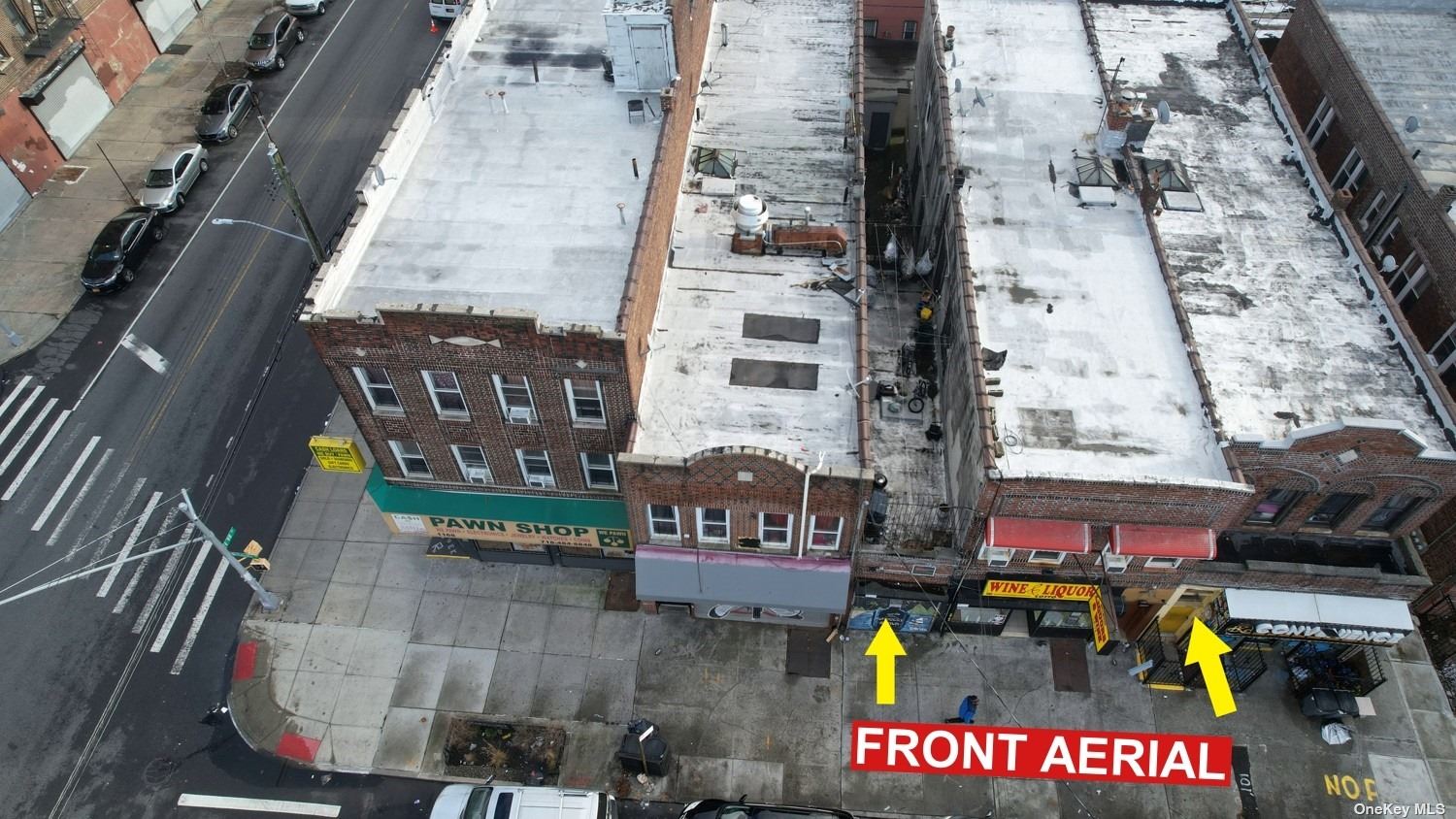This aerial color photograph captures a worn-down urban area with long, narrow buildings covered in what appears to be snow. The scene, likely taken from a drone, shows two- and three-story buildings with their facades made of brownish-reddish brick. The roofs bear air conditioning units and signs of disrepair. A busy thoroughfare runs along the left side, where cars are parked along the blacktop road. The foreground features a sidewalk lined with various businesses, including a prominently marked pawn shop and a wine and liquor store. Overlay on the image includes a red rectangular label with white text reading "front aerial" and two yellow arrows pointing towards building entrances. Despite the bustling atmosphere suggested by parked cars, none are moving, indicating a small shopping center in a less-than-desirable part of town.